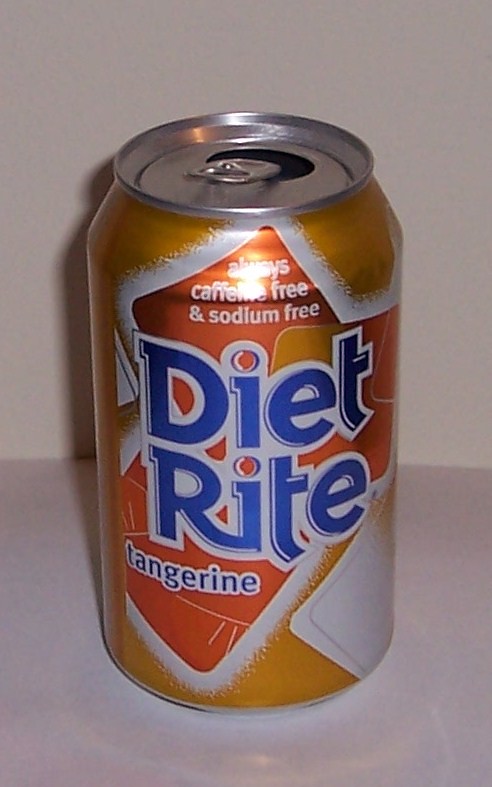This is a close-up photograph of an open Diet Right Tangerine soda can. The can, primarily featuring hues of orange with accents in white and blue, sits on a glossy, pinkish-white countertop, which subtly reflects the can’s image. The background comprises a plain, off-white wall. The soda can’s vibrant design includes different shades of orange, with the brand name "Diet Right" prominently displayed in blue letters, dotting the 'i's in red. Above this, in white letters, the can proudly proclaims "Always Caffeine Free and Sodium Free." Below "Diet Right," the word "Tangerine" is printed. The can is clean and dry, suggesting it is at room temperature and not sweating. The chrome-colored top of the can reflects additional light, enhancing the clean, crisp appearance of the metallic surface.